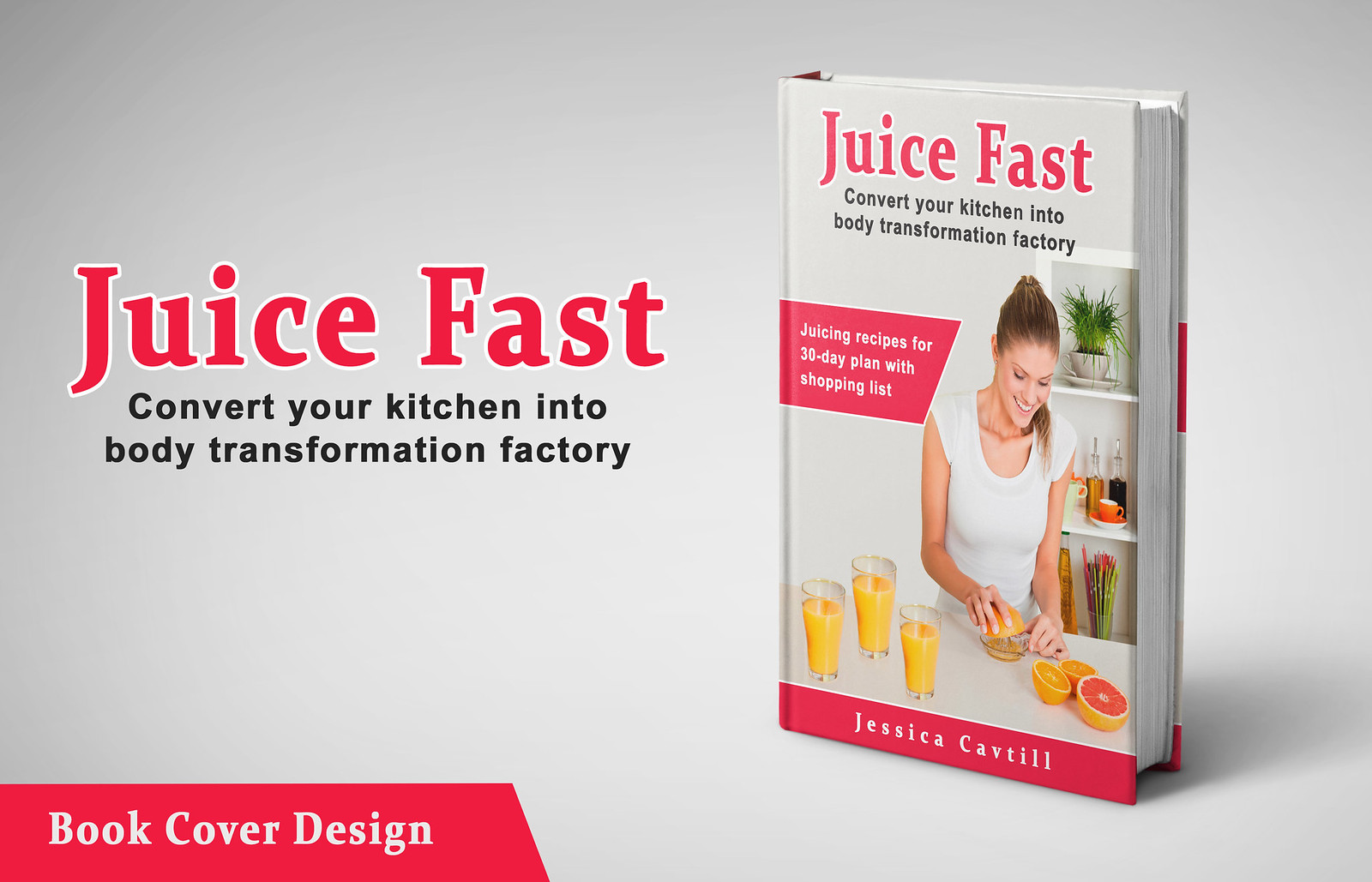This is an advertisement for a diet book titled "Juice Fast: Convert Your Kitchen into a Body Transformation Factory." The ad is set against a white and grey background. At the bottom left corner, there's a red banner with white text that reads "book cover design." Prominently displayed in large red text is the title "Juice Fast," followed by the subtitle in black text, "Convert Your Kitchen into a Body Transformation Factory."

To the right, an image of the book cover is visible. The book itself also features the title "Juice Fast: Convert Your Kitchen into a Body Transformation Factory." The cover showcases a woman, presumably the author Jessica Kevdil, who is a white woman with long blonde hair tied in a ponytail, wearing a white shirt. She is depicted squeezing oranges into three glasses of juice on a counter. The cover further highlights "Juicing recipes for a 30-day plan with shopping list," indicating it offers practical guidance for dietary planning. In the background of the book cover, a shelf with a pot of plants adds a homely touch. The author's name, Jessica Kevdil, is displayed at the bottom of the book cover within a red border. This meticulously detailed ad captures the essence and content of the book, emphasizing its transformative potential for readers' kitchens and bodies.